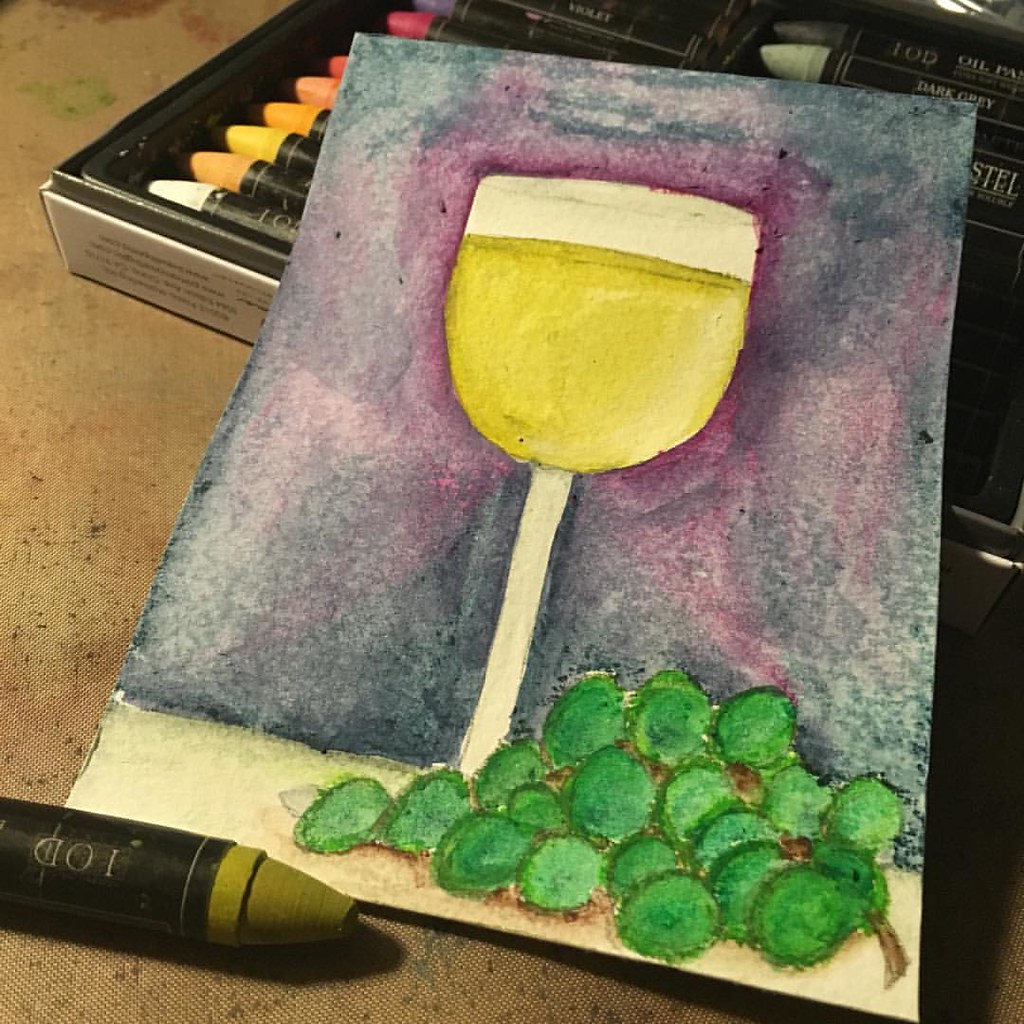This detailed close-up photograph showcases a pastel painting resting on a brown work surface that is spotted with pink and black blotches. The pastel artwork prominently features a clear wine glass containing a yellowish liquid positioned to the left-hand side of the image. On the right-hand side, a cluster of green grapes composed of many small, dark green and light green circles all attached to short round stems is depicted. The table underneath the grapes is rendered in light brown and tan hues. The background of the art piece transitions from dark blue on the edges to a rich mixture of violet and purple around the wine glass, and a purplish-dark blue blend at the base where the cylindrical stem of the wine glass meets the table.

Adjacent to the painting, there is a yellow pastel wrapped in black wax paper. Also visible in the background is a rectangular container filled with various colored pastels including shades of orange, teal, peach, white, yellow, pink, hot pink, red, purple, black, and gray. This array of pastels, lined up neatly in the box, provides a vivid contrast to the finished artwork.